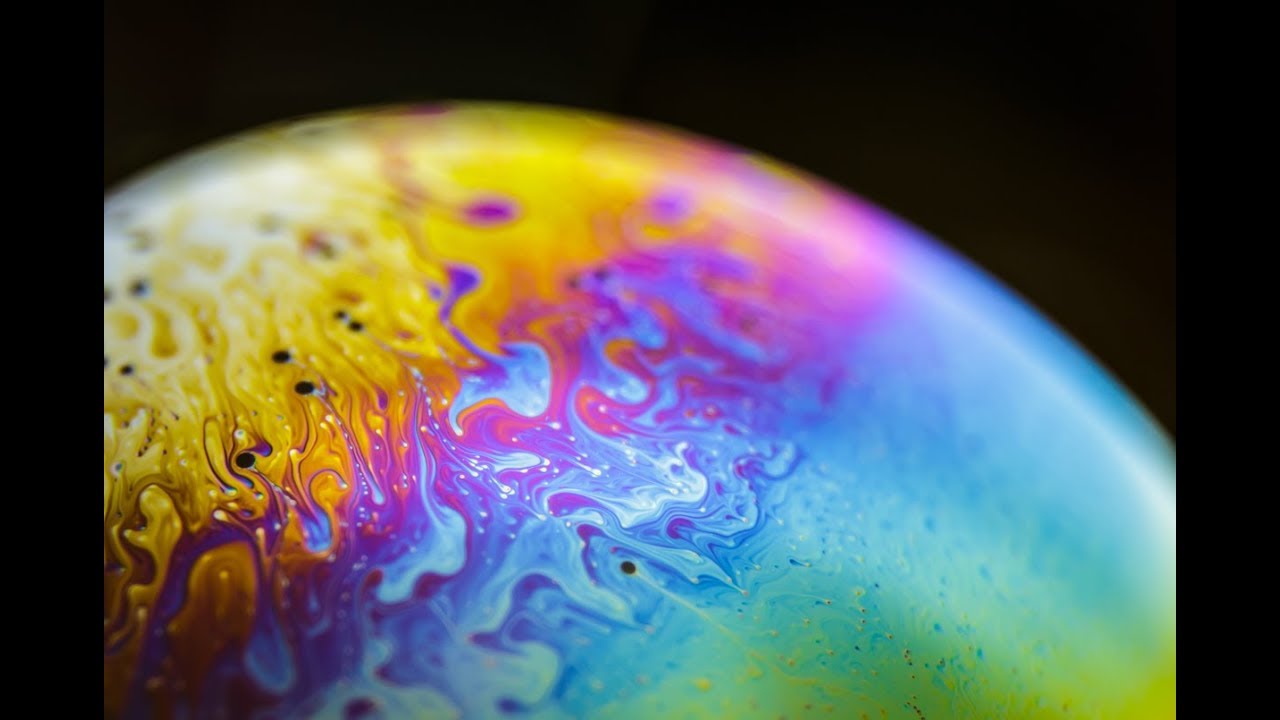This close-up image depicts a vividly colorful, ball-like sphere set against a stark black background, evoking modern artistry and leaving room for imaginative interpretation. The sphere, potentially a delicate blown glass or a digitally rendered object, is painted in a tie-dye style with colors that intricately blend and drip into one another. Accentuating a dynamic look, the top portion is predominantly yellow, transitioning through a spectrum of purple, pink, and blue, with the bottom areas showing hints of light blue, green, and a return to yellow. This vibrant mix also features cooler squiggles and dots, suggesting a wet-on-wet paint technique that allows the colors to run and meld. The shiny, glossy surface and detailed patterns add to the sphere’s striking and artistic appeal.